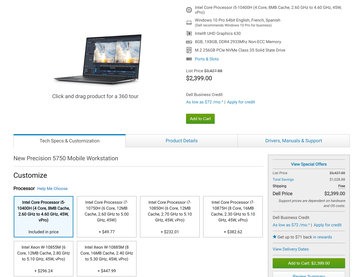**Caption:**

This image features a detailed advertisement for a Dell business desktop, powered by an Intel Core i5-10400 processor. The system boasts 8GB of RAM and comes with various customization options. The current price after applying a discount is $239. Additionally, financing is available through Dell Business Credit, offering monthly payments as low as $70.

To enhance the customer experience, the advertisement includes options for a 360-degree product tour, comprehensive tech specifications, and details on customizations. Supporting resources such as product drivers, manuals, and customer support are also highlighted. The advertisement mentions new precision bias adjustments for mobile workstations and features several offers and savings opportunities, specifying the Dell price and shipping details.